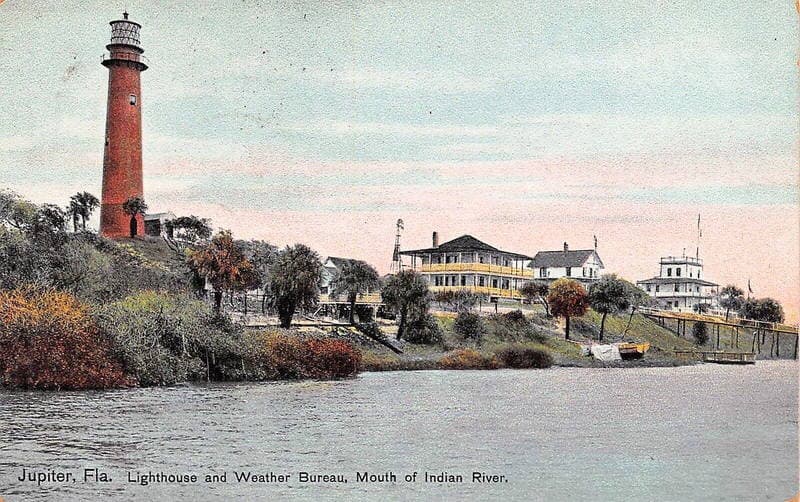This image is an old-timey, somewhat grainy painting depicting the Jupiter Lighthouse and Weather Bureau at the mouth of the Indian River in Jupiter, Florida. The scene showcases a captivating landscape with Victorian-style houses nestled along the coast of what appears to be the Indian River. In the foreground, vibrant red and yellow bushes add a splash of color beside the water, and a painted boat rests docked in the distance. The scene includes three Victorian-style beach houses, one of which has a windmill behind it. The iconic Jupiter Lighthouse, tall and red, stands prominently on a hill to the left, surrounded by several trees, completing this picturesque overview.